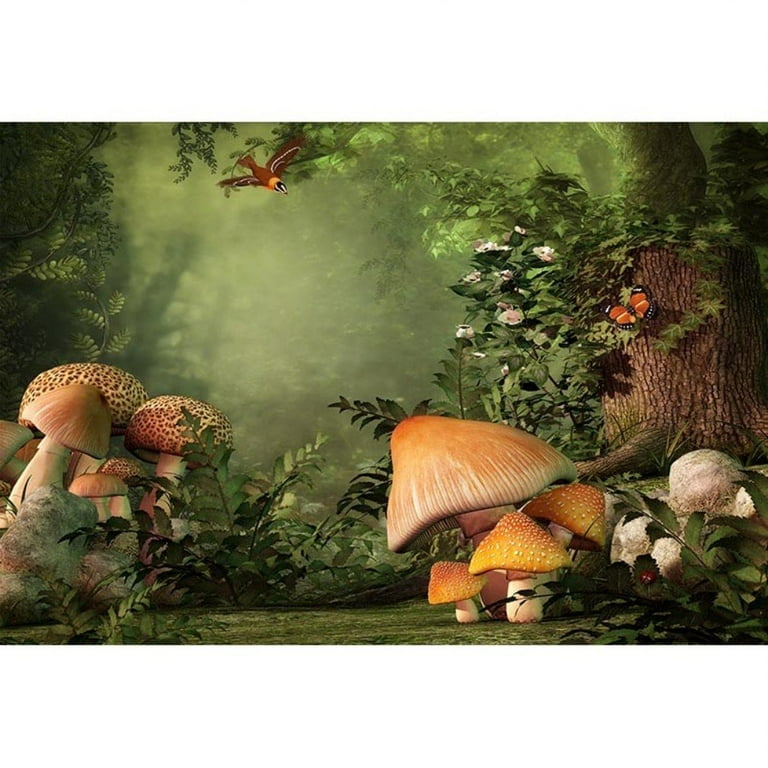The image is a highly detailed, 3D-like digital illustration of a fantastical woodland scene. It is so realistic that it almost appears photographic, capturing an enchanting atmosphere where you might expect a gnome to appear. Sunlight filters through the trees, casting a warm yellow glow in the out-of-focus background that highlights the shapes of green trees. 

In the foreground on the right side, a tree stump is entwined with ivy and adorned by an orange butterfly. Adjacent to the stump, wild roses or blackberry plants flourish, while a fern grows at its base. Nearby, a cluster of tan toadstools, some smooth and others textured with white bumps, adds to the scene’s rich tapestry. Toward the bottom right, a small red insect can be seen on the underside of another fern.

Center frame, under yet another fern, lies an additional collection of toadstools. These vary from smooth to large, rounded caps flecked with brown warty bumps. Above, a bird swoops down into the frame, adding a dynamic element to the serene setting.

Overall, the illustration is vibrant with colors and details, capturing an almost mythical and mysterious ambiance that makes it feel like a moment frozen in an enchanted forest.